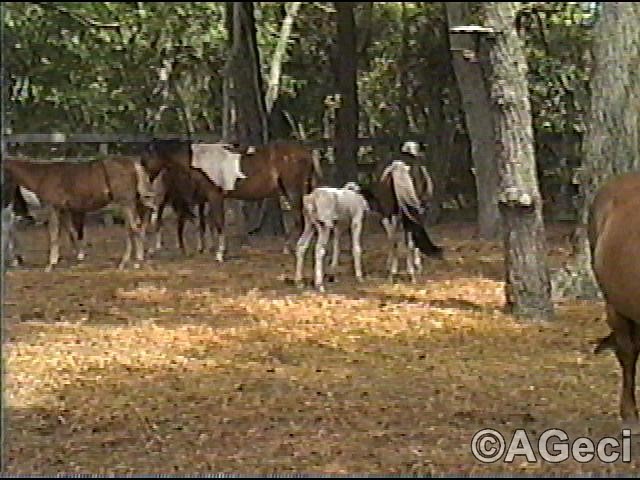The grainy, pixelated color photo, possibly taken from a digital or trail camera, depicts a blurry farm scene featuring several horses and foals in a wooden, split rail-fenced paddock. Amid the yellowish, scrubby grass and pine tree trunks, a group of horses, primarily brown with white patches, congregate. At the center, two brown horses stand in line, one slightly obstructed from view, each looking to the left. A foal, white in color, stands between these horses, back turned to the camera, appearing to nurse from a mare. The mare, characterized by white legs and a tail with both white and brown hues, stands to the foal's right. Light filters through the trees, casting dappled patterns across the pen, while the lower right corner of the image bears a watermark reading "© AGECI," with "A" and "G" in uppercase and "ECI" in lowercase.